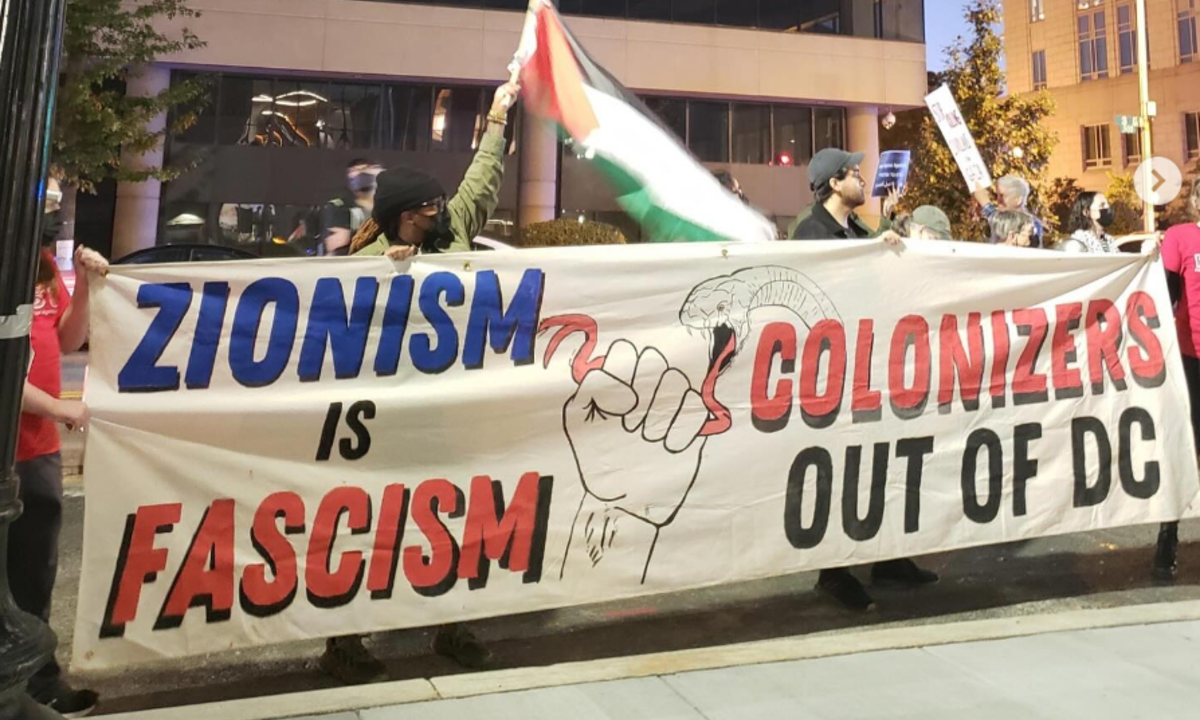This photograph captures a vivid scene of a street protest, where a diverse group of demonstrators stands unified in front of a sidewalk, holding a substantial white banner, approximately 15 feet long. The banner is emblazoned with the statement "Zionism is Fascism" — 'Zionism' written in bright blue, 'IS' in black, and 'Fascism' in bold red letters. At the center of the banner, there's a striking image of a monochrome fist gripping the tongue of an illustrated snake. To the right, the words "Colonizers out of DC" are boldly displayed, with 'Colonizers' in red and 'out of DC' in black. Among the protesters is a man on the left, notable for his army green shirt, black hat, and goggles. He is holding a Palestinian flag, which is red, black, green, and white. The determined and serious expressions on the protesters' faces are palpable, and many are wearing masks and various types of headwear, underlining the gravity and solidarity of the demonstration.